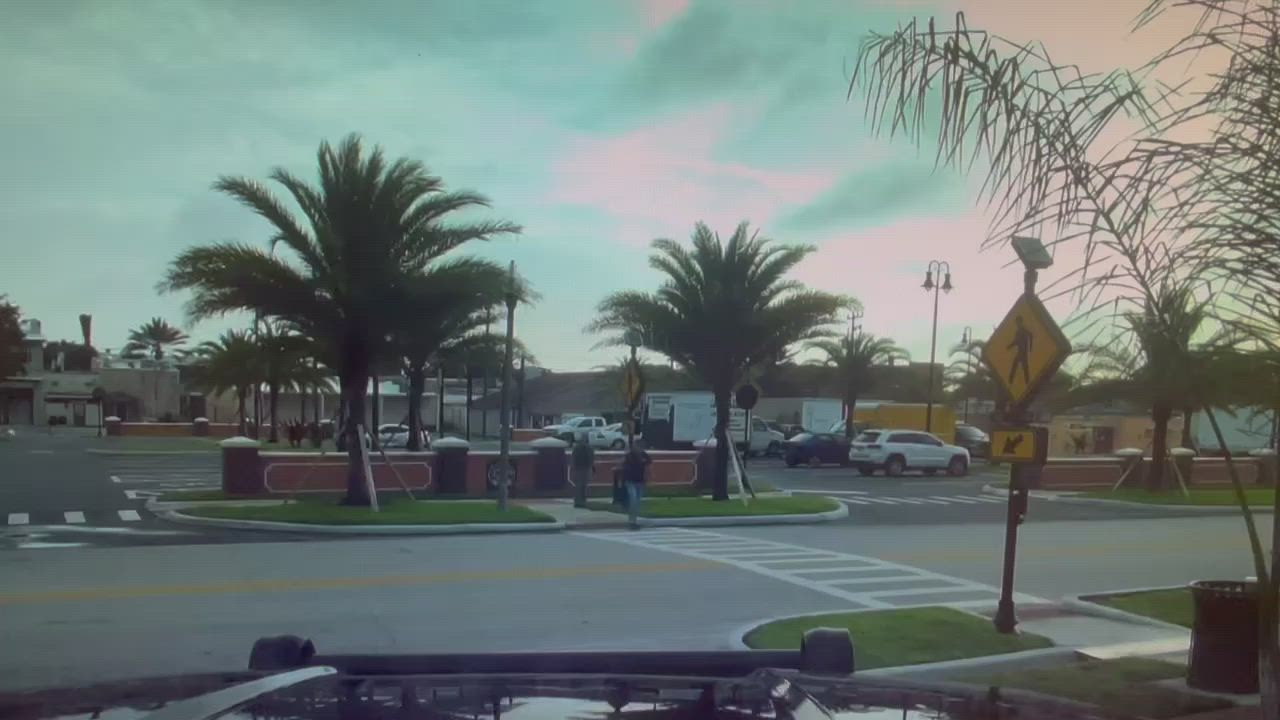This vibrant color photograph captures a roadside scene featuring a variety of elements. Dominating the center of the image are a tall palm tree and a smaller one, standing against a reddish-brown wall with a patch of green grass at their base. To the right, a road intersects with a clearly marked pedestrian walkway, denoted by white lines. A yellow pedestrian crossing sign with a black figure is positioned near the left corner of the image. At the bottom of the photograph, a long, rectangular dark grey object is visible, possibly the inner edge of a vehicle. The sky above is a unique bluish-green shade, contrasting with the foliage. In the upper right corner, some fern-like trees frame the scene, while a few cars are faintly visible in the background, slightly to the right of the palm trees.